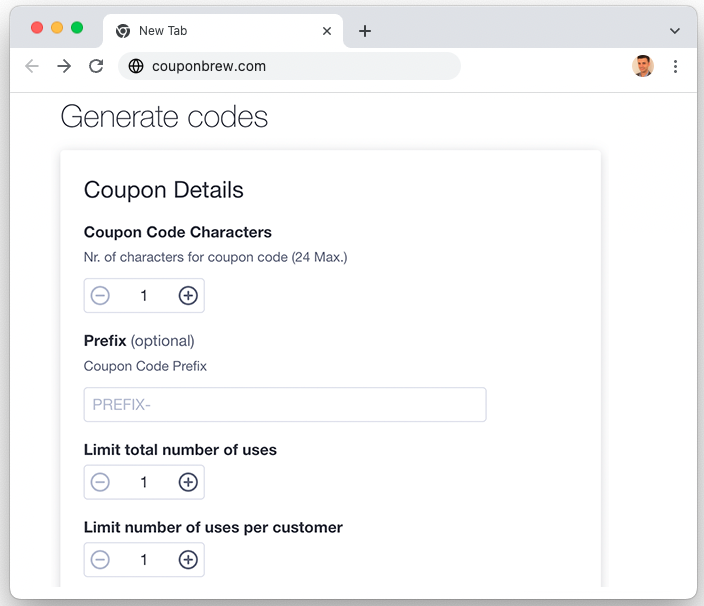A person is using a Chrome browser on a Mac desktop or MacBook. This is evident because the browser displays the distinctive Mac minimization, maximization, and exit buttons on the top left corner, represented by the red, yellow, and green dots, respectively. 

The URL bar is a prominently elongated oval shape, featuring a small gray globe icon on the left side, indicating that the current website is 'couponbrew.com'. To the right of this URL bar, there is a small user icon with a beige background depicting a man with light brown hair. Next to this icon, there are three vertically aligned dots, signifying a dropdown menu.

Beneath the URL bar, a light gray divider separates it from the content below. The visible text below the divider reads "Generate Codes". Following this, there's a square menu area with the header "Coupon Details" in bold font. Just below this, in a smaller but bolder font, it states "Coupon Code Characters." Further down, in smaller gray text, it reads "Nr. of characters for coupon code (24 max.)."

Below this text, there is an option to change the quantity of something, featuring a minus sign within a circle on the left and a plus sign within a circle on the right. The minus sign is disabled and shaded light gray, indicating it’s inactive because the current selection is set to one, allowing only an increase.

Directly beneath this selection tool, there is a header labeled "Prefix" in bold, with the word "optional" next to it in parentheses and non-bold gray text.